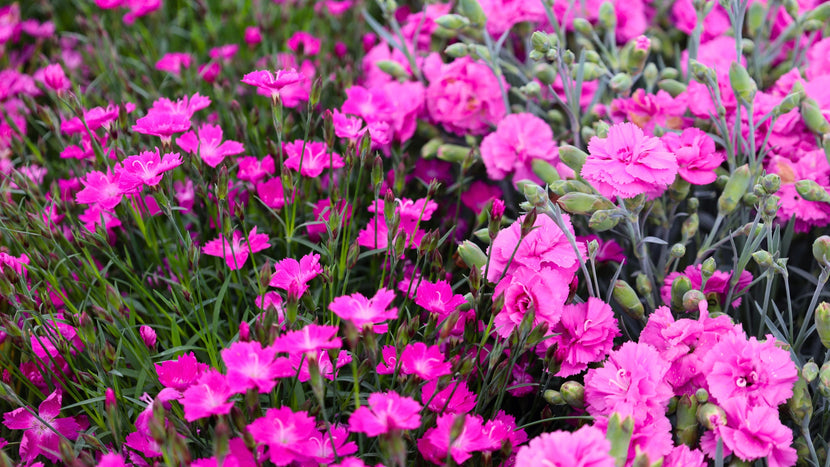This is a vibrant, color photograph showcasing a zoomed-in view of a field adorned with blooming pink flowers. The majority of these flowers resemble roses, with broad, multi-petaled, furled pink blooms that dominate the image. Interspersed among these are another variety of pink flowers that feature a distinctive white center and a prominent, slightly hooked white protrusion. Some of the flowers are still in bud form, presenting as small, green, unopened blooms. The scene also includes visible stems and green blades of grass that weave through the floral display, emphasizing the flowers' natural, field setting. The petals of the flowers range in color from bright pink to hot pink, with many flowers fully open, adding to the overall lushness and vividness of the image.